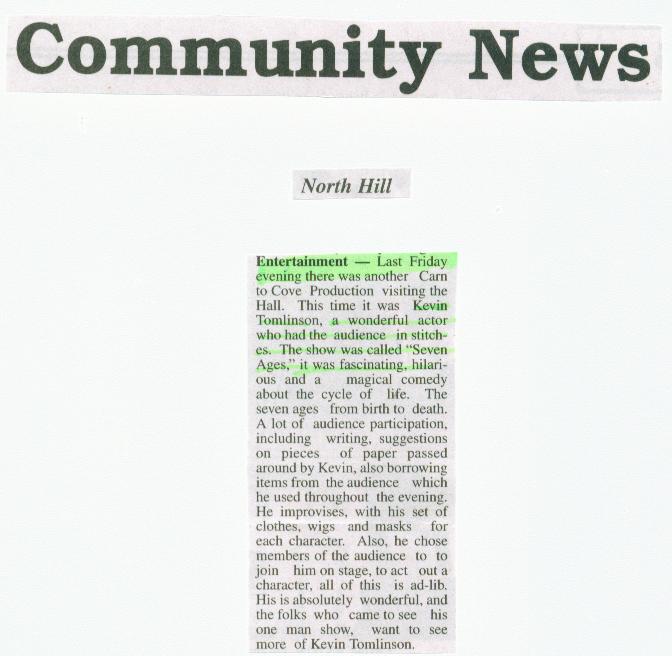The image features a newspaper clipping glued onto a white background, possibly an A4 sheet. At the top, it says "Community News" followed by "North Hill." The main newspaper snippet, highlighted in sections with a green marker, details an entertainment event. It reads: "Last Friday evening, there was another Corinda Cove production at the hall. This time, it featured Kevin Tomlinson, a wonderful actor who had the audience in stitches with his show 'Seven Ages.' The performance was fascinating, hilarious, and magical, depicting the cycle of life from birth to death. Tomlinson's one-man show involved a lot of audience participation, including writing suggestions on slips of paper and borrowing items from the crowd. He skillfully improvised using a variety of clothes, wigs, and masks to portray different characters, even inviting audience members to join him on stage. The overall reaction was overwhelmingly positive, with attendees eager to see more of Tomlinson's captivating performances."